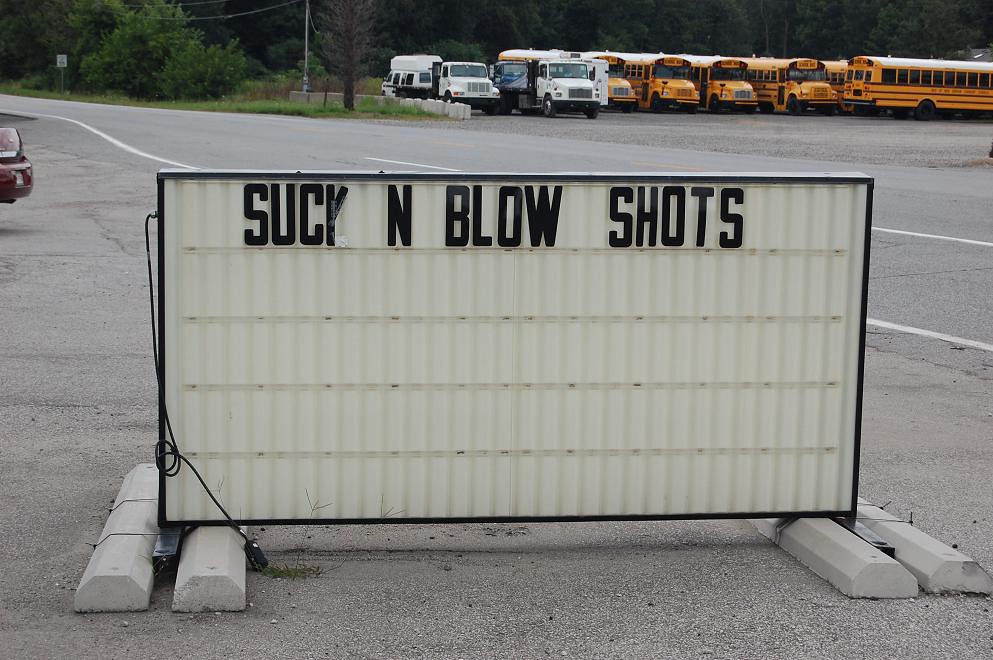The photograph depicts a large white billboard with a black frame, prominently situated just off a two-lane asphalt road, likely in a rural or backwoods area of America. The main focus of the image is this backlit sign, held upright by two sets of concrete blocks on either side to prevent it from tipping over. The text on the sign, displayed in black capital letters, reads "SUC N BLOW SHOTS." Notably, the lower part of the letter "K" is missing, making it appear as "SUCY" initially. In the background, the scene reveals a parking lot filled with six or seven yellow school buses and a couple of white work trucks with black beds, along with a white Dodge camper van situated in the top right corner. A bank of trees lines the background, adding a touch of greenery to the setting. The edge of a car bumper encroaches on the left-hand side of the image, further emphasizing the roadside location.